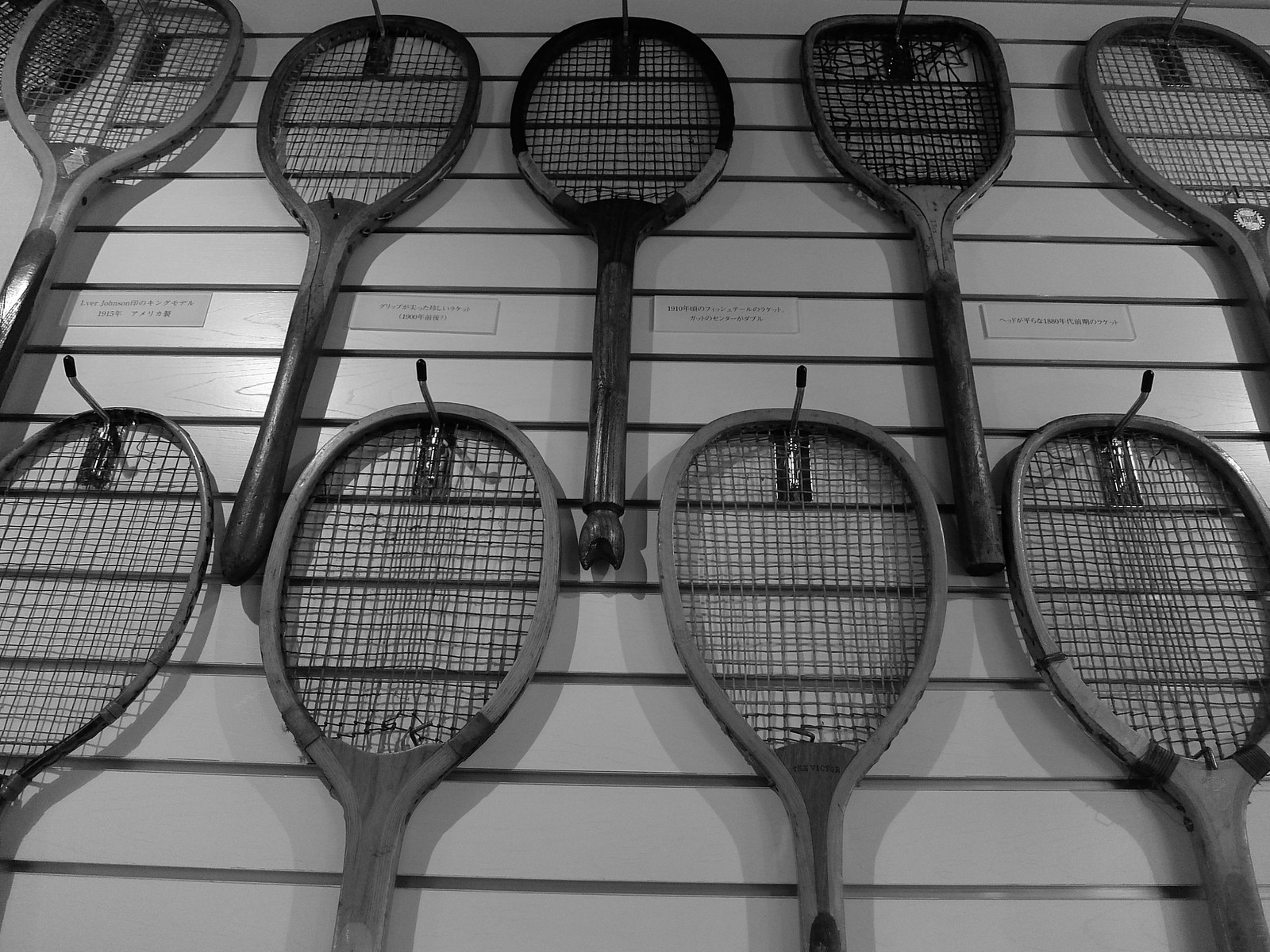The black-and-white photograph captures an artistic arrangement of vintage tennis rackets against a vertically paneled wooden wall, painted gray. Taken from a low angle, the image reveals two rows of rackets, the top row featuring five while the lower displays only the tops of four. Each racket hangs from a black-tipped silver hook. The rackets have dark or possibly black handles, though it's difficult to ascertain exact colors due to the monochrome aesthetic. Some have black tape wrapped around certain areas and small rectangular pieces of paper with undecipherable text, possibly in Japanese, Chinese, or English, identifying the rackets. A notable racket in the top row diverges with a spatula-like shape, adding variety to the otherwise oval and circular collection. Shadows cast across the scene suggest slightly underexposed lighting, enhancing the vintage feel of the meticulously composed frame.